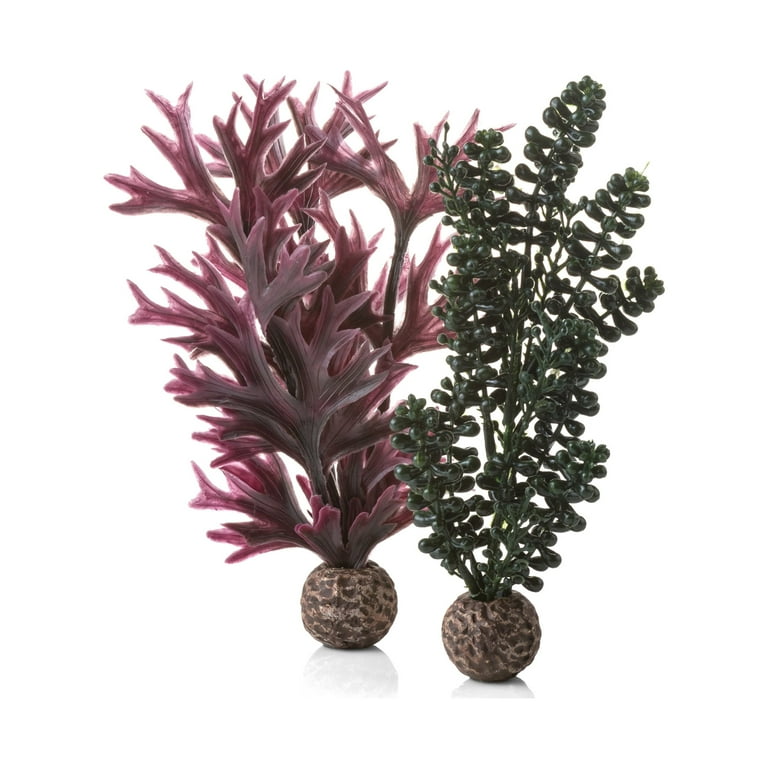This minimalist image features two artificial plants set against a stark white background. Each plant emerges from a small, spherical container that resembles a textured stone with brown indentations on a goldish-tan surface. On the left, a visually striking plant boasts dark purple, antler-like appendages with pointed tips, extending in various directions and resembling intricate neural dendrites. To the right stands an equally striking artificial plant, characterized by dark green, teardrop-shaped leaves that appear bulbous and somewhat firm. Both plants, similar in height at approximately six inches, offer a sharp contrast against the simplicity of their white surroundings, allowing their unique forms and vibrant colors to dominate the scene.